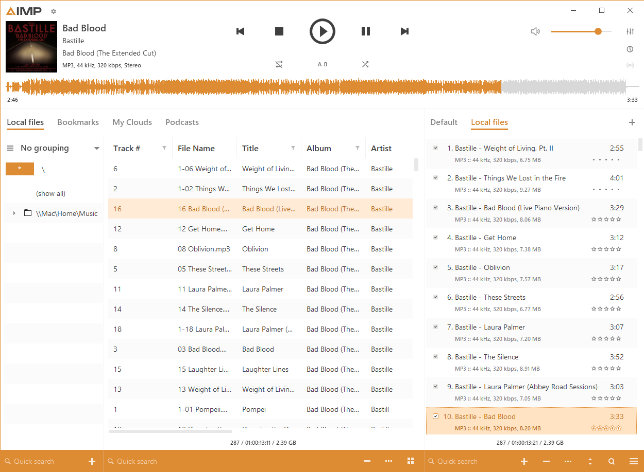A screenshot of a desktop music player called "Imp" is displayed. The interface is somewhat blurry but reveals a wealth of details. The player appears to be currently playing Bastille's album "Bad Blood," specifically the extended cut version. The audio quality is noted as 320 Kbps in stereo. Traditional media control icons are present, including play, stop, fast forward, rewind, and volume control, along with a volume meter.  

At the bottom center of the interface, various tabs are visible, labeled "Local Files," "Bookmark," "My Clouds," and "Podcasts." A list of tracks from the "Bad Blood" album is partially visible, including "The Weight of Things," "Oblivion," "These Streets," "Laura Palmer," "The Silence," "Bad Blood," "Laughter Lines," "Weight of the Living," and "Pompeii."

The file structure indicates that the software is running on a Mac, as evidenced by the "Mac Home Music" label at the top-right section of the screen. Below this, another list of local files includes several Bastille tracks: "Weight of the Living," "Things We Lost in the Fire," "Bad Blood," "Get Home," "Oblivion," "These Streets," "Laura Palmer," and "The Silence.” Some tracks appear multiple times.

On the bottom section of the interface, there's a small star icon for favoriting tracks. Also visible in orange are a quick search button and additional plus and minus icons, suggesting options for further navigation or organization. Overall, this appears to be a desktop music organizer tailored for detailed music file management.